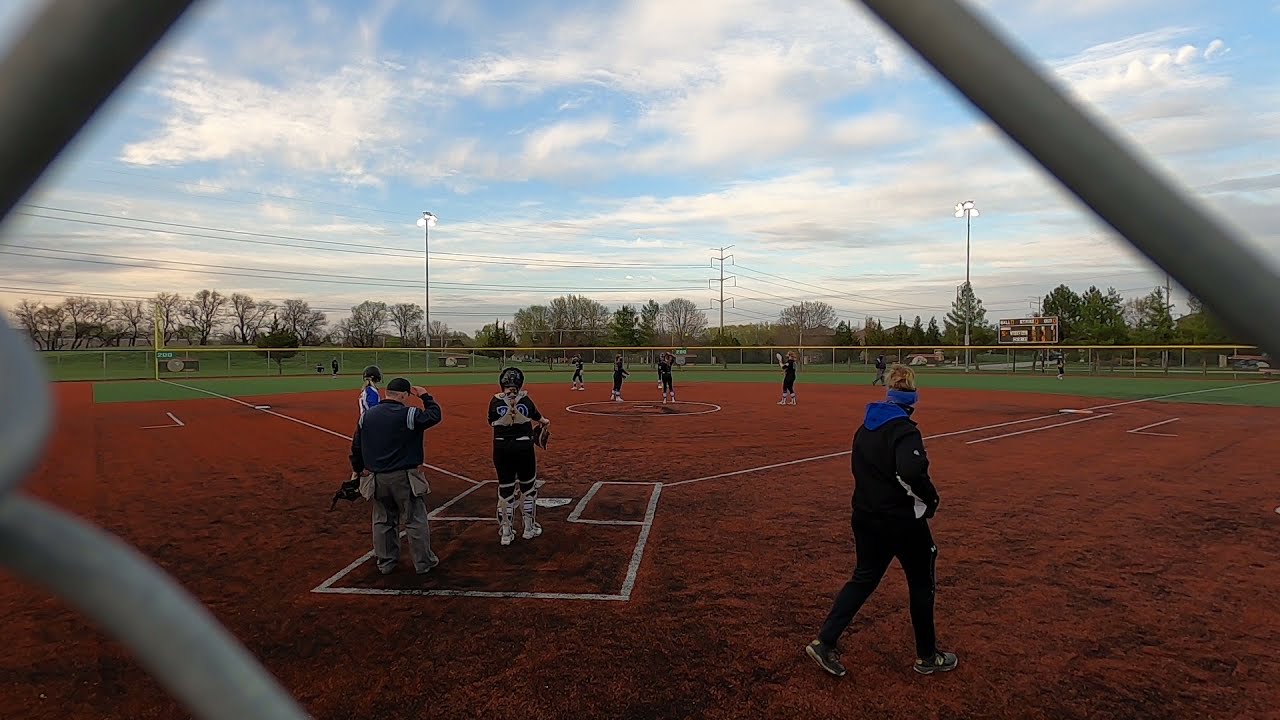This photograph captures a vibrant baseball game in progress from an intriguing perspective, taken behind a metallic fence. The wide rectangular image provides a full view of the baseball field, with the reddish-brown diamond in the foreground marked by white lines. The grassy outfield appears lush and green, bordered by a metallic fence. In the background, several tall electrical poles and power lines stretch horizontally across the image, interspersed with numerous trees, some fully leaved and others bare. The sky overhead is a bright blue, dotted with several white, wispy clouds. 

In the lower right corner, a woman with blonde hair, dressed in black sweats, walks across the scene carrying what appears to be a clipboard. Near her stands an umpire adjusting his cap, and further left, a player readying himself for the game. Additional players are scattered across the field, standing in the outfield in anticipation as the game is about to commence. To the right of the field, a scoreboard is visible, along with tall stadium lights. The photograph aptly captures the lively, detailed environment of a daytime baseball game.